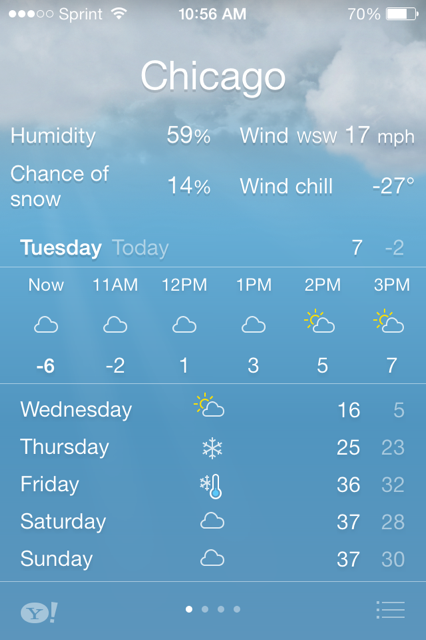This detailed caption describes a screenshot of the Apple Weather app. The top bar shows a series of three to five dots partially filled in, indicating signal strength, with "Sprint" as the carrier and a Wi-Fi symbol to its right. The time is displayed in the center as 10:56 a.m., and the battery level shows 70% with a respective icon on the right. 

The background of the Weather app screenshot transitions from blue at the bottom to cloudy at the top. "Chicago" is prominently displayed in white text. Additional weather details include 59% humidity, a west-southwest wind blowing at 17 miles per hour, a 14% chance of snow, and a wind chill making it feel like -27 degrees. The day is Tuesday, with a forecasted high of 7 degrees and a low of -2 degrees for the day.

Below this, a timeline provides hourly temperature updates:
- "Now" showing a cloud icon with -6 degrees
- 11 a.m. with a cloud icon indicating -2 degrees
- 12 p.m. with a cloud icon showing 1 degree
- 1 p.m. with a cloud icon displaying 3 degrees
- 2 p.m. with a sun-behind-cloud icon at 5 degrees
- 3 p.m. with a sun-behind-cloud icon at 7 degrees

Further down, the app displays the upcoming weather forecast:
- Wednesday: Sun-behind-cloud icon, high of 16 degrees, low of 5 degrees
- Thursday: Snow icon with a high of 25 degrees, low of 23 degrees
- Friday: Snow icon behind a blue thermometer (indicating low temperature) with a high of 36 degrees and low of 32 degrees
- Saturday: Cloud icon with a high of 37 degrees and low of 28 degrees
- Sunday: Cloud icon with a high of 37 degrees and low of 30 degrees

At the bottom of the screenshot, icons are visible that suggest the ability to swipe for additional information.